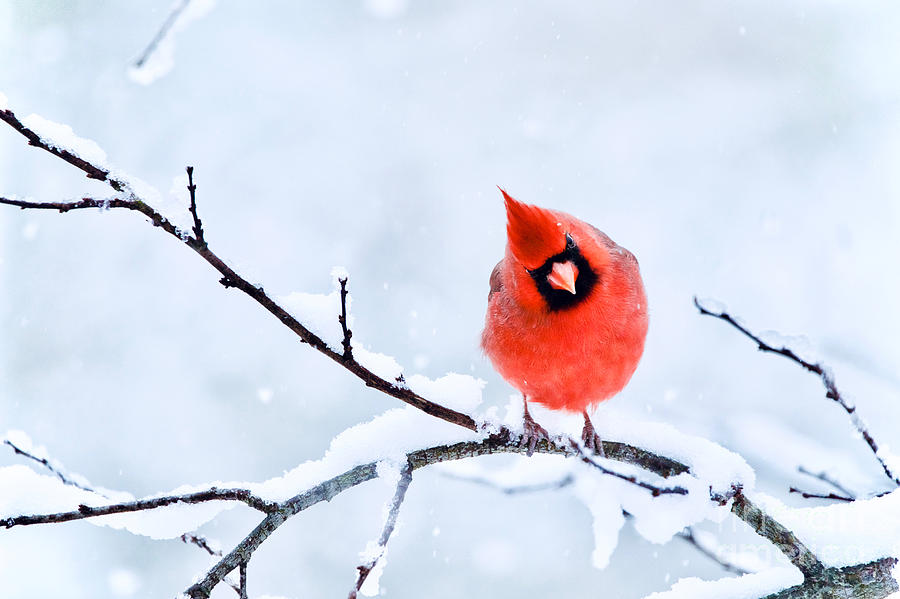This photograph features a vibrant male cardinal perched on a snow-covered, gray tree branch in a serene winter scene. The bright red bird, positioned slightly right of center, stands out against the grayish-white, icy blue background, which suggests a recent snowfall. The cardinal's distinct black square mask extends from one eye to the other, framing its reddish beak that pierces through the snowy ambiance. Both of the cardinal's feet grasp a small branch that emerges from the bottom right corner of the image; this branch bends slightly under the bird's weight and forks just beyond its feet. One twig from the fork stretches toward the upper left, while the other bends downward, with a multitude of smaller twigs branching off. The cardinal's head is tilted to the left as it looks directly at the camera, capturing an intimate and striking portrait of nature's resilience and beauty amidst the cold.